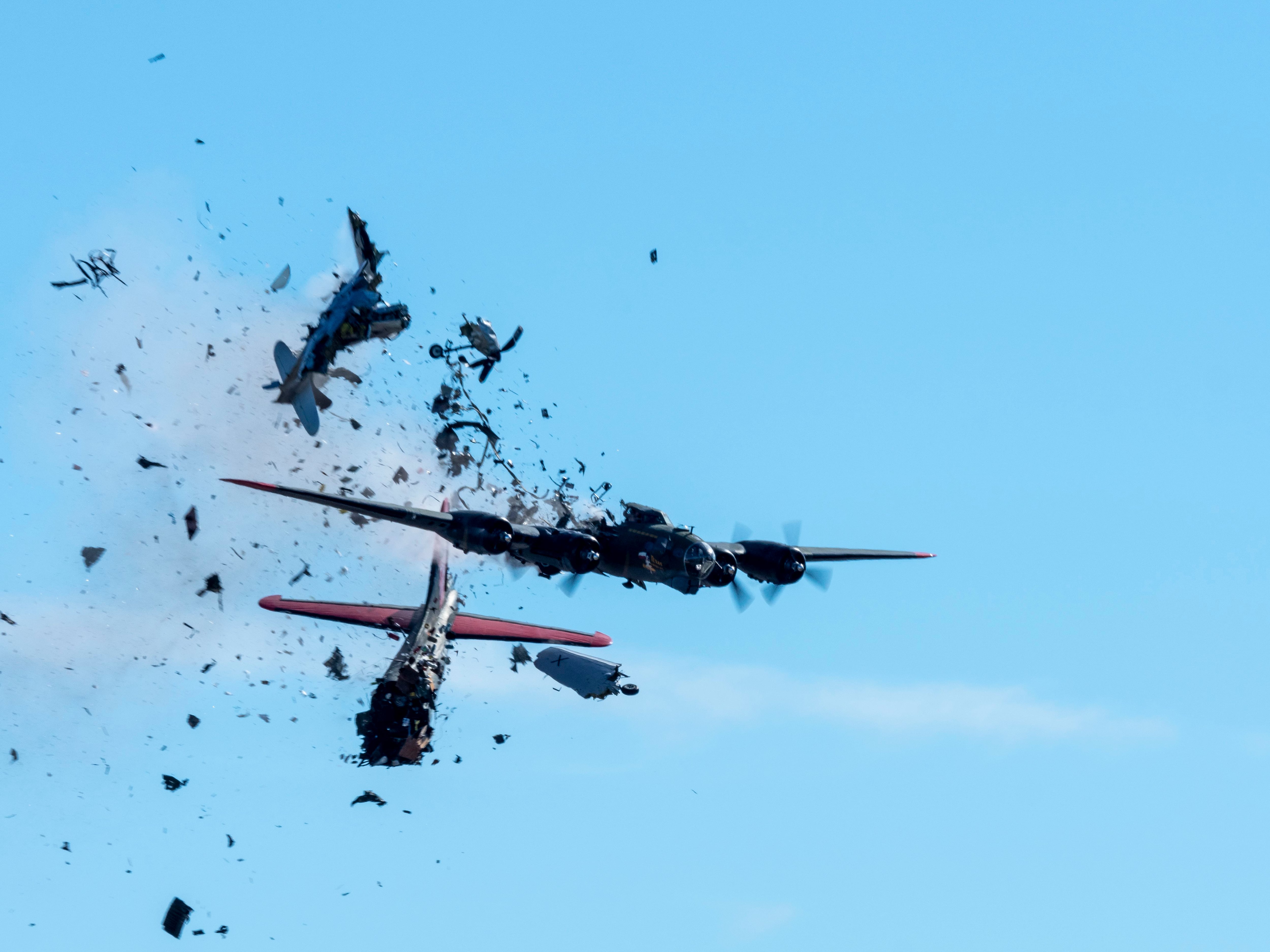The image captures a dramatic scene of a mid-air collision involving two aircraft against a light blue, almost cloudless sky. Central in the image is an airplane, oriented as if flying towards the viewer, with its right wing and propeller still intact and in motion. The back of this plane is obliterated, with fragments trailing behind it. Below and slightly to the left of the main plane, another aircraft, seemingly a military fighter plane, is caught in mid-descent. This second plane is also ravaged by the impact, with its rear wings and part of its body still visible, but the front part is missing, and debris falls around it. The chaotic scene is punctuated by a scattering of debris and smoke, conveying the violence of the collision. The remaining sections of both planes, along with the visible spinning propellers of the first plane, add to the graphic depiction of this aerial disaster.